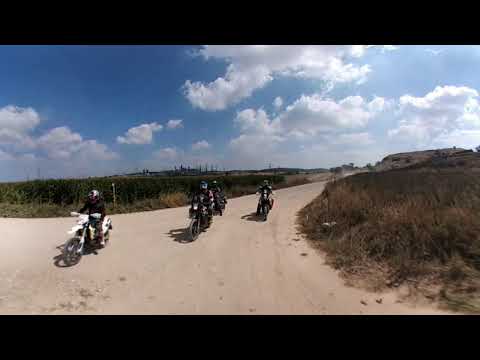In this low-quality image, we can see a group of four dirt bikers traveling along a sandy, light tan dirt road. The dirt road is framed by tall, greenish-brown grass on both sides, interspersed with weeds. Particularly notable is the lush, farm-field-like greenery on the left-hand side, contrasting with the slightly wilder vegetation on the right, leading into a mountainous backdrop. The sky above is a deep blue, filled with large, thick white clouds, creating an overcast effect. The dirt bikers are positioned centrally in the image, with the closest rider on a white bike clearly visible on the left side. The remaining three bikers' details are obscured. The image is bordered by horizontal black bars at the top and bottom, similar to widescreen borders, adding to the compressed and artifact-laden quality of the picture. No text is present in the image, and the overall setting suggests it was taken outdoors in the middle of the day on a dirt bike path.